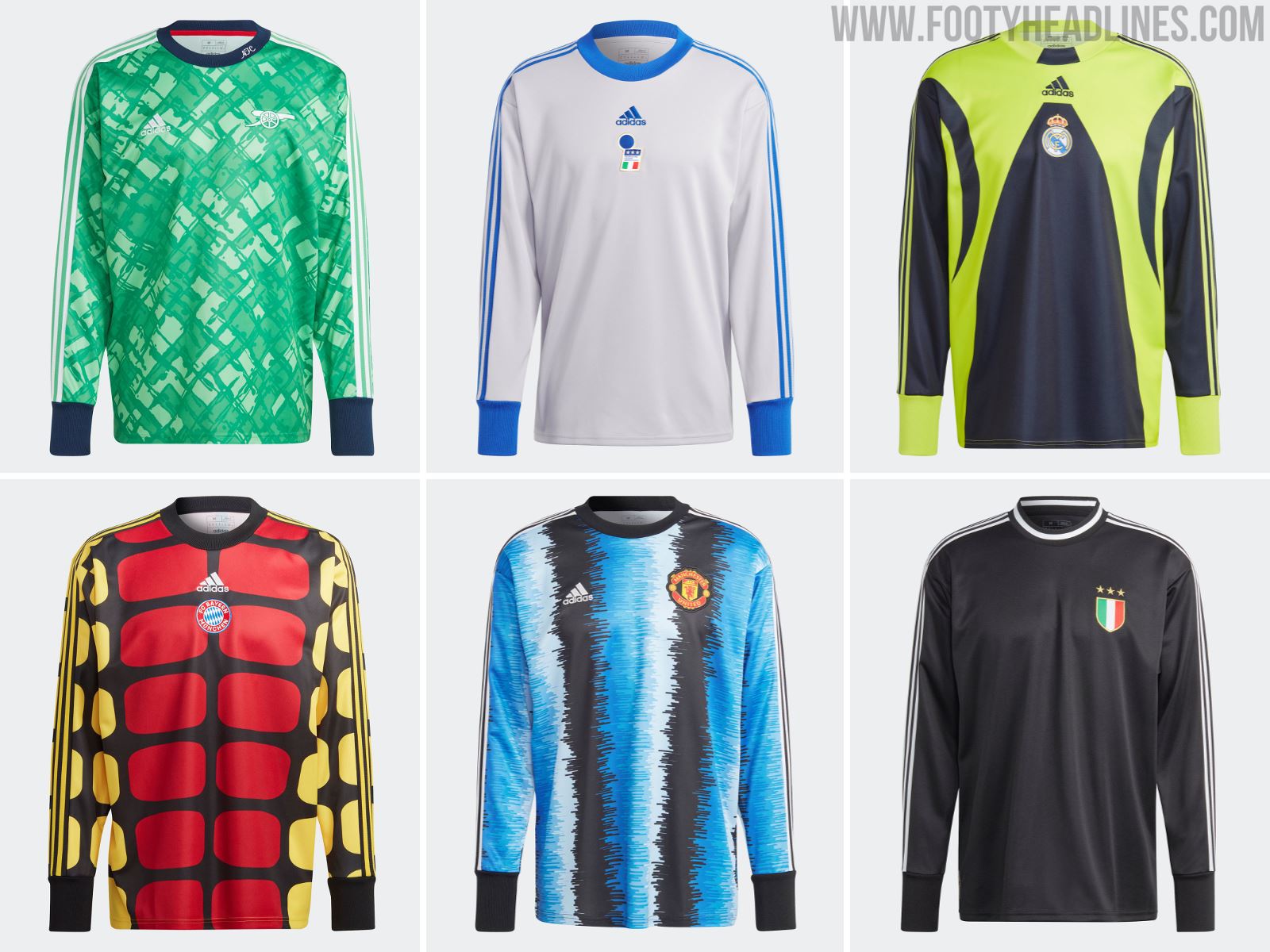In the composite image, six distinct styles of long-sleeve athletic shirts are displayed, each housed in its own rectangular frame. These jerseys, likely designed for soccer, feature unique color schemes and patterns, predominantly branded by Adidas, with various team logos.

Starting from the top left, the first shirt is a vibrant green with navy cuffs at the sleeves and white stripes running down the arms, paired with a blue collar. The second shirt, next to it, is white adorned with blue stripes on the sleeves and a matching blue collar. It bears the Adidas logo and a small flag beneath it.

The third shirt, placed at the top right, showcases a striking black and white design, highlighted with neon yellow accents forming a triangular pattern emerging from the bottom center. This jersey also includes the Adidas logo and a team crest.

Shifting to the bottom row, the fourth shirt on the far right is another predominantly black design, featuring white stripes on the sleeves and topped with an Italian flag crest on the chest. To its left, the fifth shirt displays a dynamic pattern of black, white, and sky blue stripes, contributing to a tie-dye effect.

Lastly, the sixth shirt on the bottom left commands attention with its bold primary colors: red dominating the center framed by yellow on the sleeves and sides, bordered by intricate black webbing. Each of these jerseys embodies distinct team aesthetics, tailored for pre-game warm-ups.

The branding is consistent across most jerseys, with Adidas prominently displayed and an additional website URL, www.bootyheadlines.com, noted in the top right-hand corner of the image.